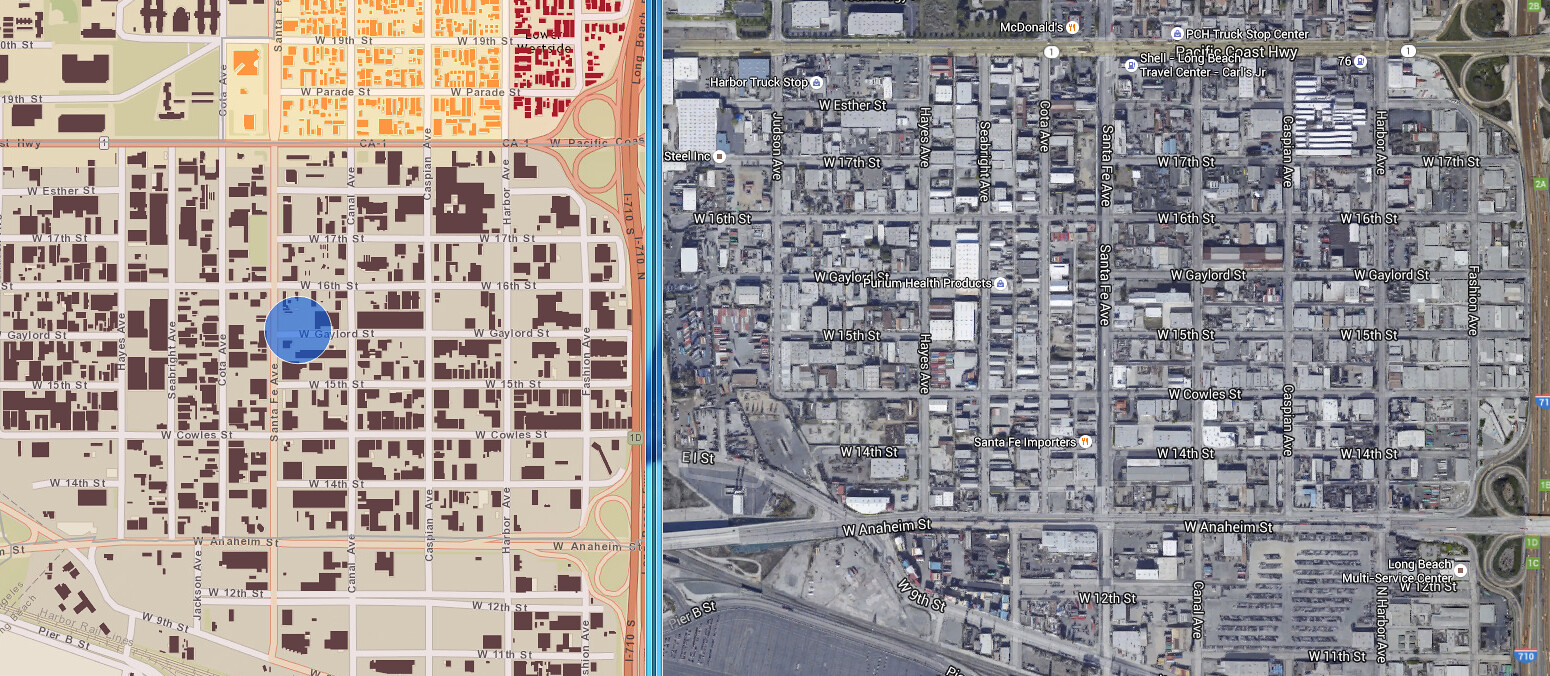This image shows a complex city map, seemingly generated from a mapping program. The map is divided into two distinct sections: the left 40% is rendered in a series of flat colors, denoting different types of zones and properties. Prominent markers in this section include yellow spots indicating houses or properties, with additional red and brown markers designating other notable areas. Centrally within a densely brown-marked area around West 16th Street, a blue dot signifies the location of the map user.

The right 60% of the image portrays a continuation of the city but in black and white, creating a stark contrast and suggesting either a division within the same map for different viewing purposes or perhaps the juxtaposition of two separate maps. The overall map covers a dense urban environment filled with numerous houses, buildings, industrial zones, and freeways. This section of the city appears intricately detailed, highlighting the hustle and complexity of urban life.